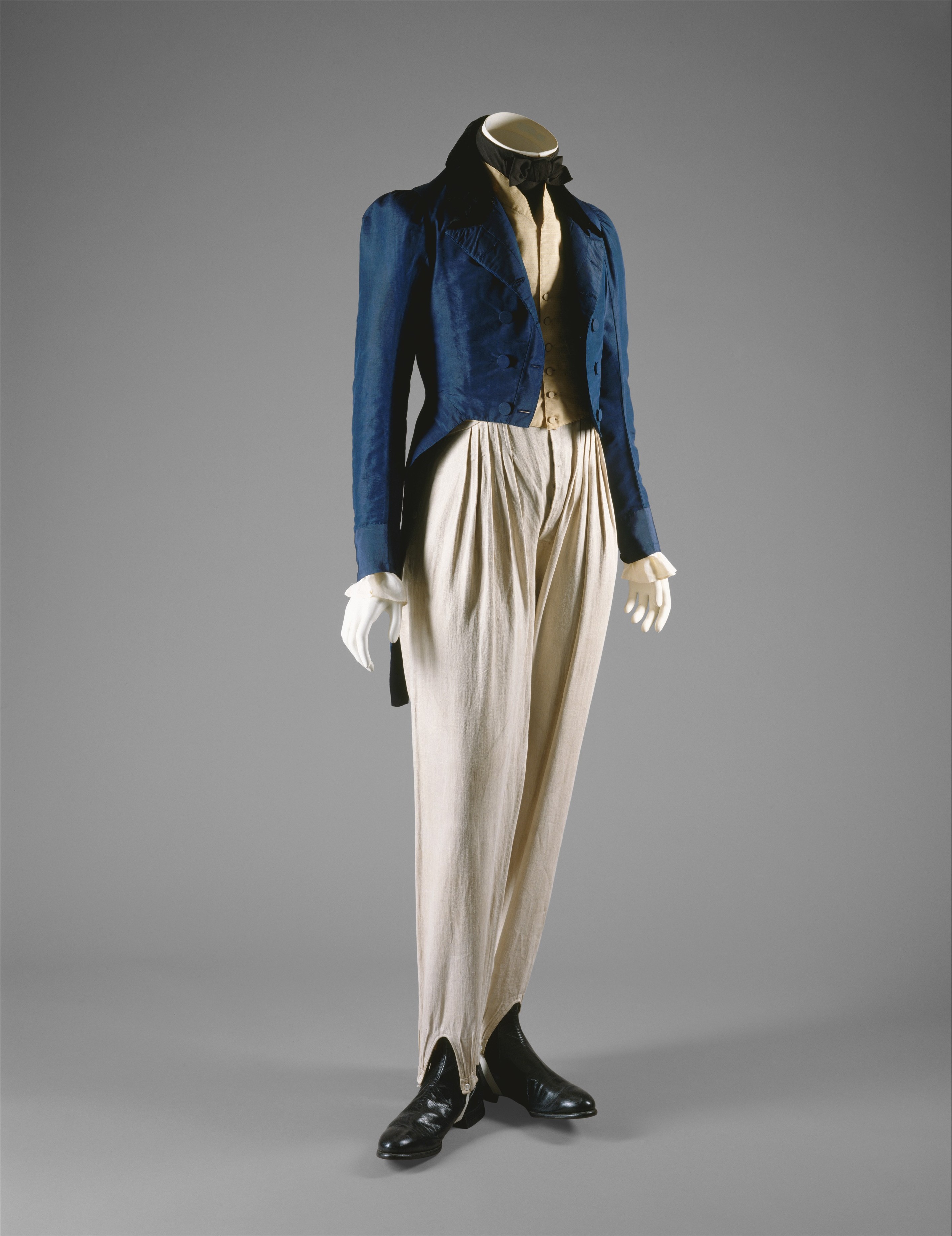The photograph features a headless white mannequin dressed in an elaborate, vintage men's outfit, evocative of the 1800s era. The ensemble includes a pair of black leather boots with white pantaloons made from canvas or cotton material, secured with straps around the boots. The mannequin wears long white pants and a beige or tan vest, buttoned up over a white shirt with frilly, fluffy cuffs extending out of the sleeves of an unbuttoned blue waistcoat. A black bow tie or neckerchief adorns the neck, completing the sophisticated look. The entire display is set against a seamless gray background and floor.